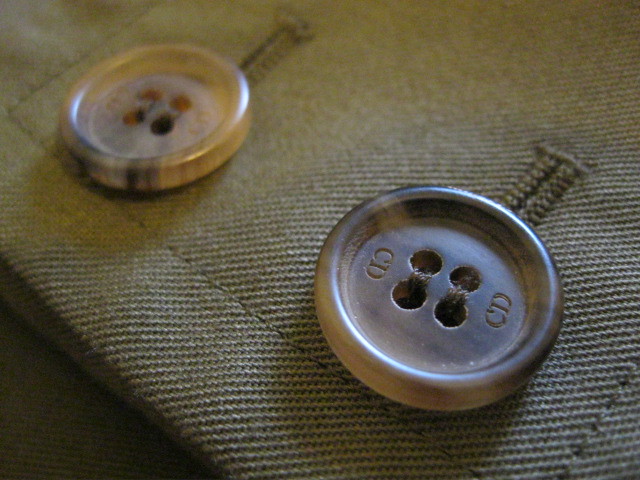This close-up photograph captures two brown buttons on what appears to be a houndstooth-patterned jacket. The fabric displays a rich texture with detailed stitching, reminiscent of a thick, well-crafted material. The foreground features a slightly larger, more prominent button in focus, embossed with "CD" on either side of its four holes, through which red thread is intricately sewn. Just above this button, the edge of the buttonhole seam is visible, adding depth to the image. The second button, slightly more beige and out of focus, lies behind the first, appearing smaller due to the angle of the shot. Both buttons share similar characteristics and display the meticulous stitching that secures them firmly to the fabric.